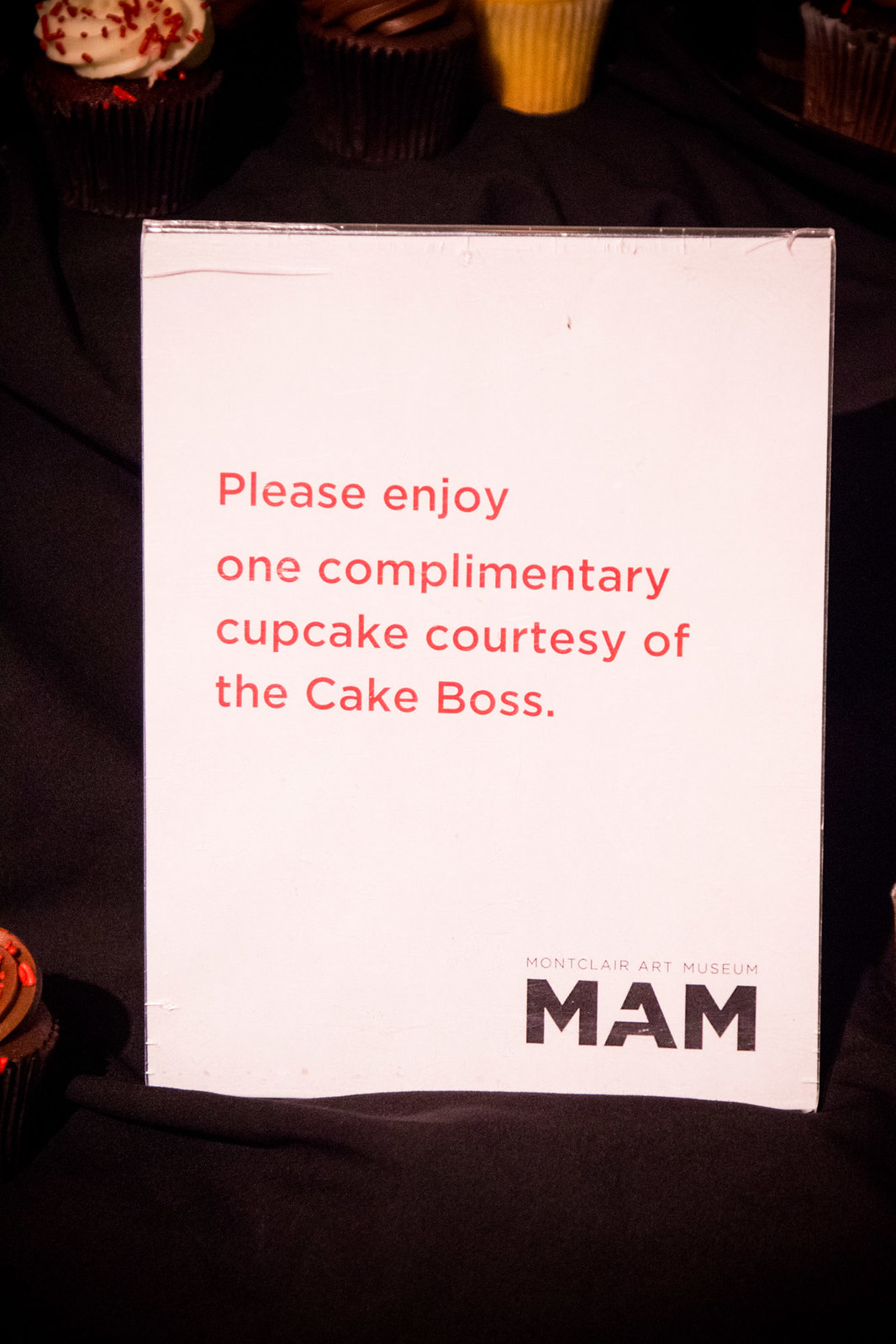The image features a small white sign against a black background, likely from an event. The sign reads, in red letters: "Please enjoy one complimentary cupcake, courtesy of the Cake Boss." Below this, in very tiny text, it mentions "Montclair Art Museum" and below that, in larger black letters, it shows the museum's logo, "MAM." Positioned near the top left corner of the sign is a cupcake with white frosting and red sprinkles, partially visible. Next to it are another chocolate cupcake and a vanilla cupcake. The lower left corner of the image also displays a cupcake with brown icing.